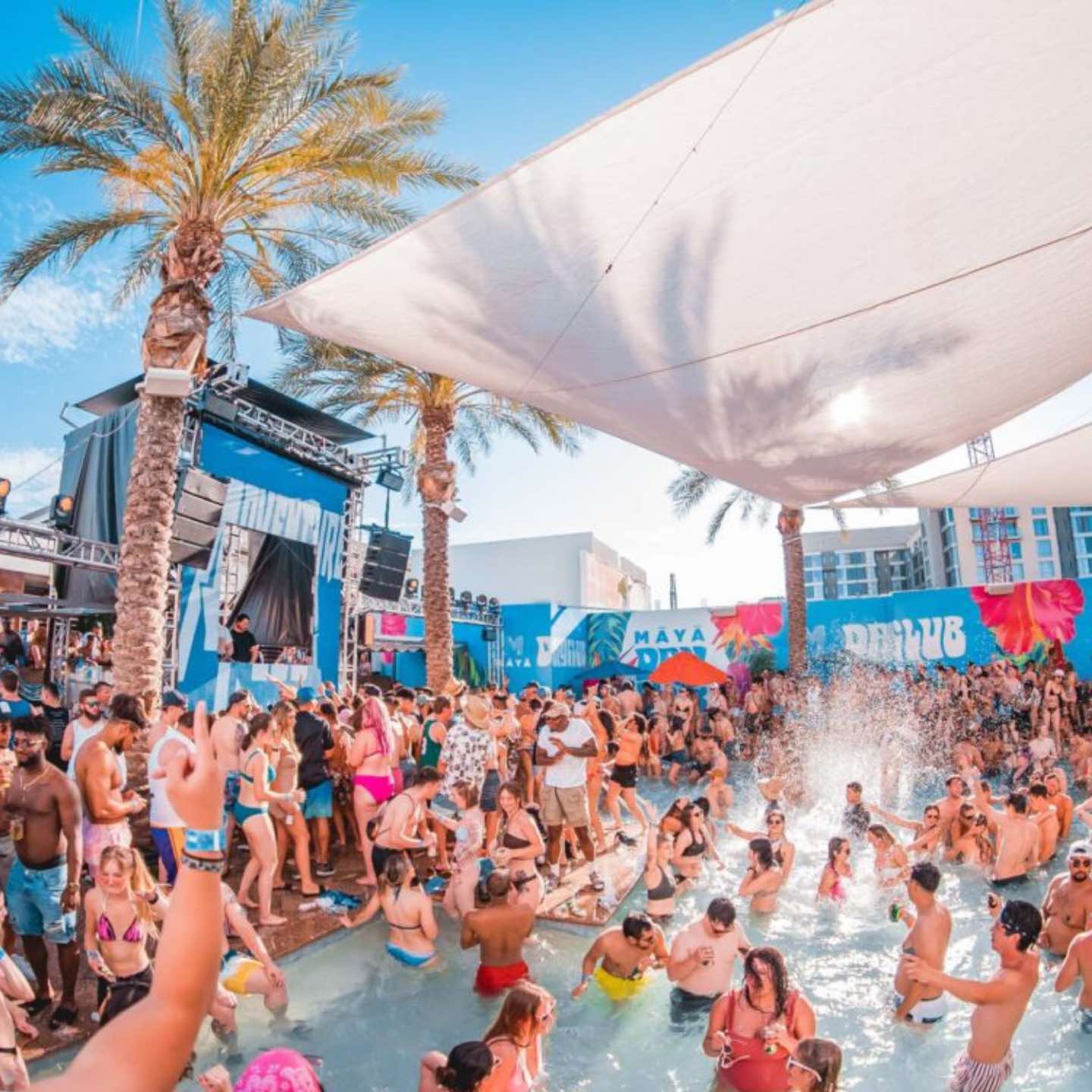The photograph captures the vibrant scene of a spring break party at a beach resort. In the foreground, a large, shallow swimming pool is teeming with people enjoying the festivities, some cooling off in the water while others splash and play. Men are shirtless, wearing swim trunks, and women don an assortment of colorful swimsuits. Several party-goers hold drinks as they celebrate in the pool. Surrounding the pool, additional revelers stand and walk around, adding to the lively atmosphere. A white awning, tied to the tops of palm trees, provides some respite from the sun as it stretches over the pool. To the left, a concert stage or DJ booth outlined in bright blue, pink, and orange hues adds a musical backdrop. In the background, multi-story hotels and buildings with windows rise against a clear blue sky dotted with a few clouds. A blue fence adorned with red flowers runs along the perimeter, enhancing the festive environment. Overall, the scene is one of carefree enjoyment under the palm trees and open sky, epitomizing the essence of a spring break celebration.